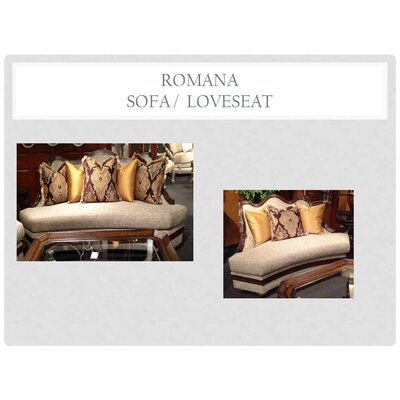The image prominently features a luxurious sofa labeled "ROMANA" in black, all-caps font, situated at the top-center over a white background. Below, it says "SOFA / LOVESEAT," also in black, all-caps font within a white rectangle, all set against a gray backdrop. The sofa boasts an elegant design with a gray base and wooden accents framing the piece and a slightly wavy backrest. The first image, positioned in the top left of the gray box, presents a direct, frontal view showing five patterned cushions: a central cushion in gold and burgundy, flanked by two gold cushions, with another pair of patterned cushions on either side. The secondary image, to the right, offers a side perspective, revealing the same cushion arrangement and the wooden frame.